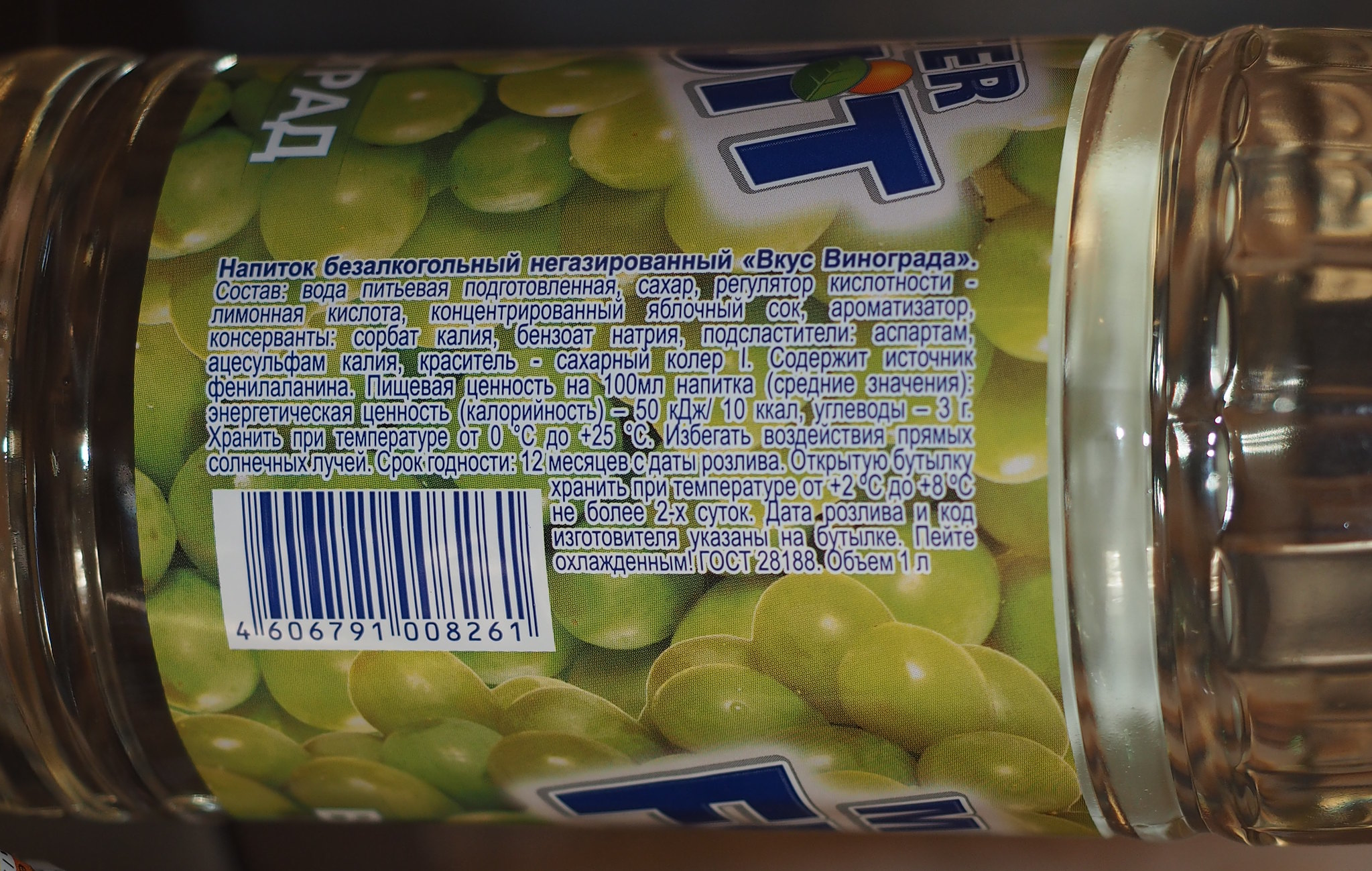This horizontal close-up image features a glass jar with its lid sealed and positioned to the right. The jar, possibly photographed in a kitchen setting, showcases a label adorned with green olives or similar fruits. The label is predominantly in dark blue with a striking white outline, making the foreign text, potentially Eastern European or Russian, stand out. This text likely includes ingredient information. Prominently placed at the bottom left of the label is a white barcode with blue lines, displaying the numbers "4-606-791-008261." At the top part of the label, the letters "E, R, and T" are partially visible, while at the bottom, the letters "F and M" can be discerned.